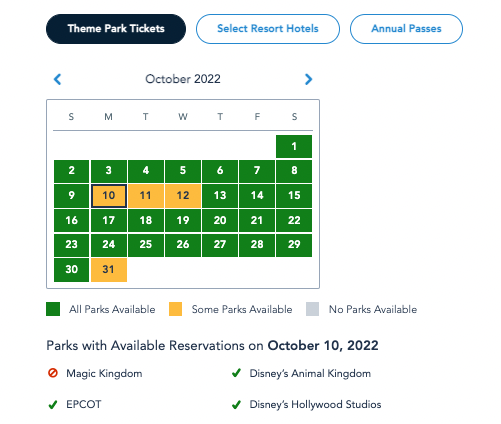This screenshot displays a reservation system for a theme park. At the top of the interface, there are three navigation buttons: "Theme Park Tickets," which is currently highlighted, "Select Resort Hotels," and "Annual Pathways," both of which are not highlighted. Directly beneath these buttons is a calendar for October 2022. 

The calendar includes a left arrow to navigate to September and a right arrow to navigate to November. The days of the week (Sunday through Saturday) span across the top, followed by individual dates from 1 to 31. The dates 10, 11, 12, and 31 are highlighted in yellow, indicating that "Some Parks Available" on these days, while the remaining dates suggest that "All Parks Available." There are no dates marked with "No Parks Available."

Below the calendar, there is a section labeled "Parks with Available Reservations on October 10, 2022." It lists the availability status for each park:
- Magic Kingdom: Not Available
- Epcot: Available
- Disney's Animal Kingdom: Available
- Disney's Hollywood Studios: Available

This captures all the information presented on this page.